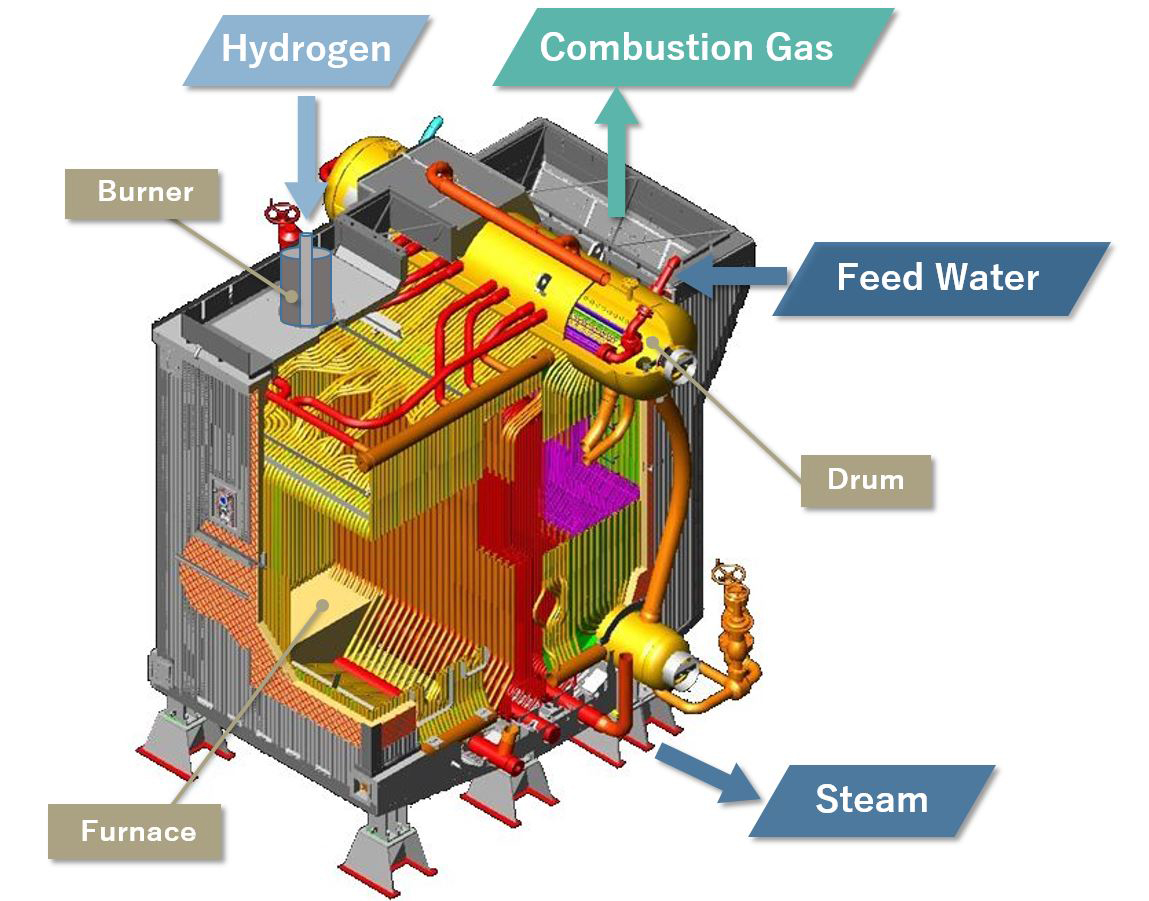The image appears to be a detailed, labeled diagram of a furnace, possibly intended for educational purposes or as part of an instruction manual. The diagram is illustrative with a white background and the outer casing of the machine rendered in a gray metallic color. The furnace has an overall square structure with approximately four to five silver peg feet at its base, providing support. The outer layer of the furnace is cut away to reveal the complex internal components, which are vividly colored in bright neon shades including red, green, yellow, orange, and pink. Numerous wires and pipes inside the machine are color-coded for easy identification.

Key components of the furnace are clearly labeled with arrows pointing to their respective parts. Labels include "hydrogen," "combustion gas," "burner," "feed water," "drum," "furnace," and "steam." The label "furnace" is found at the bottom left, with an arrow leading to the center of the machine. The label "burner" is at the top, followed by "hydrogen" which points downward into the assembly. "Combustion gas" is labeled on the right side, directing attention to the corresponding part inside. Continuing around, "feed water," "drum," and "steam" labels are positioned towards the bottom right, each with arrows indicating their specific locations and functions within the machine. The diagram’s use of bright colors within the machine's interior and a monochromatic metallic exterior helps to distinguish between different parts and their paths, making it functional for understanding the complex workings of the furnace.